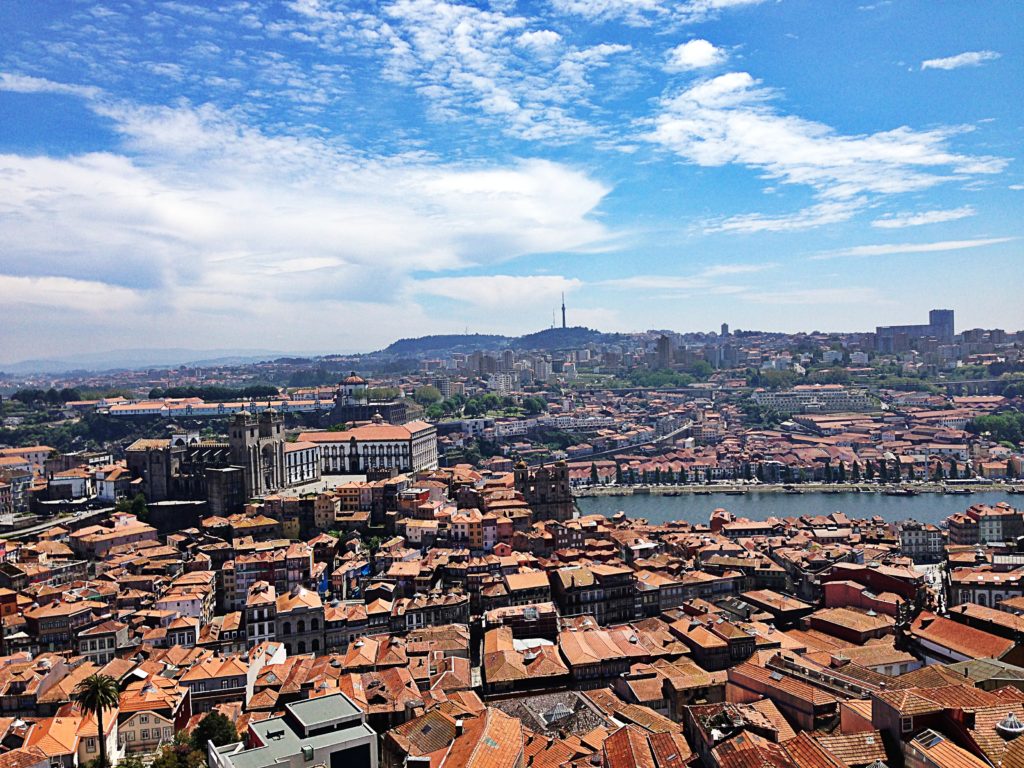An aerial view captures a sprawling, historical European city with an intricate maze of reddish clay-tiled rooftops interspersed with a few gray-roofed buildings. The bottom half of the image is dominated by these older structures that nestle closely together, evoking the appearance of a bustling hive. On the right side of the image, a wide river courses through the urban landscape, lined with trees and possibly resembling the Thames or other significant European waterways. A dock is visible at the far end of the water. The left side prominently features a grand cathedral with two towers flanking a central archway and what might be a dome structure nearby. In the background, tall hills rise up with a small tower perched atop the central hill, all under a canopy of blue skies dotted with clouds, hinting at a serene yet storied environment.